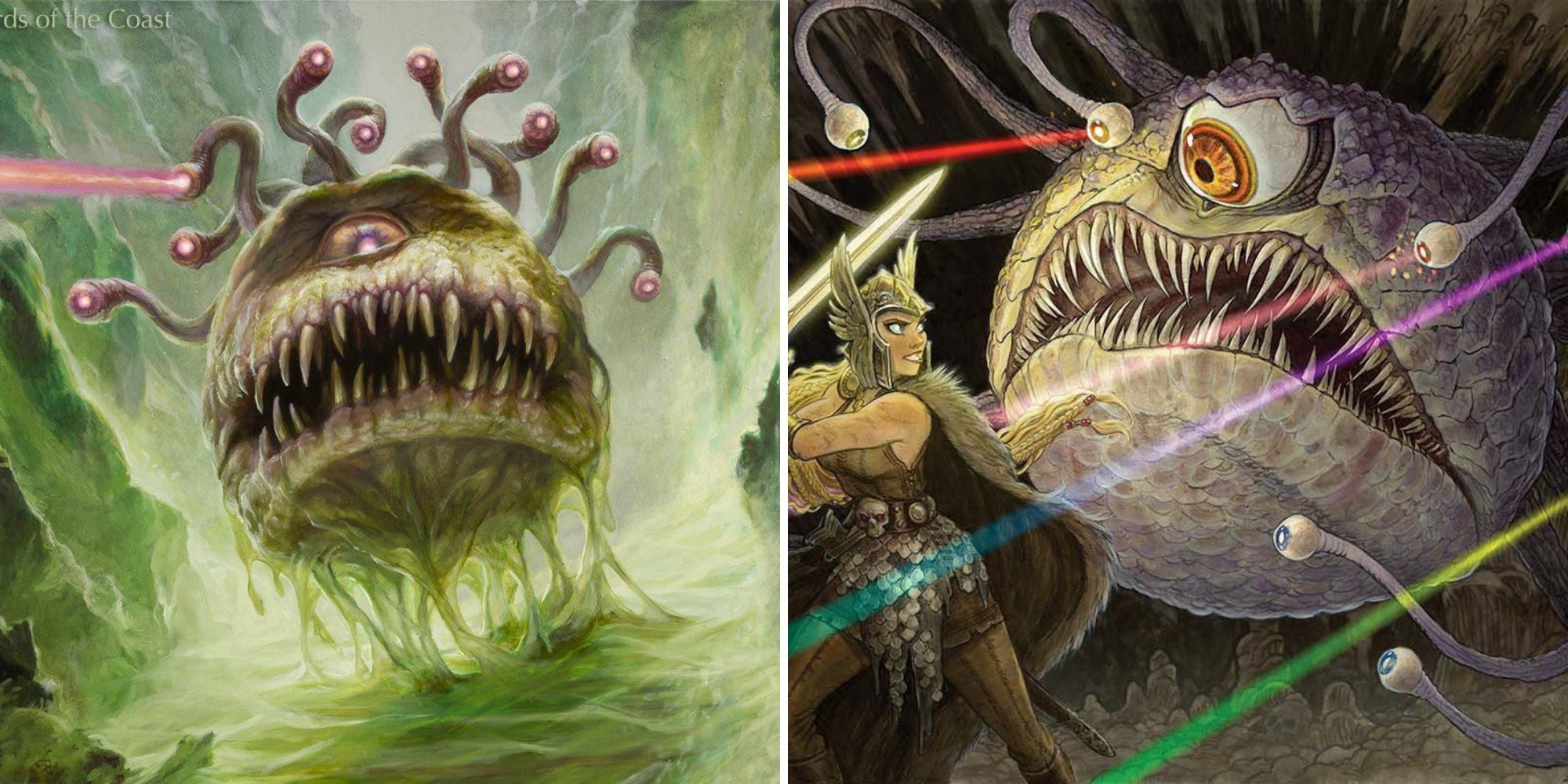The image consists of two panels depicting a fantastical creature and a fierce battle. In both panels, the creature—a giant, one-eyed monster—is featured prominently. It has a spherical body covered in green slime, with a massive, gaping mouth filled with hundreds of sharp teeth that span from edge to edge, resembling a shark's maw. The monster's head is adorned with numerous tentacles, each ending in what appears to be an eye, from which laser beams of various colors shoot out.

In the left panel, the creature is shown in what seems to be a cave, surrounded by green rock walls and a river of green slime. The atmosphere is eerie with the predominant hues of green creating a ghastly backdrop, possibly illuminated by the creature’s own bioluminescence.

The right panel shifts the scene to a more dynamic and cartoonish depiction, where the same monstrous being faces off against a Viking-like warrior woman. The woman is geared for battle, wielding a sword and clad in a helmet with feathers, a fur cloak over her shoulders, and a skirt that appears to be made of snakeskin. Her ensemble is completed by tan pants and a belt adorned with skulls. The creature’s expression shifts to one of concern as it engages in combat, with its tentacles actively shooting beams of red, purple, and green-yellow light. The environment remains filled with green, wave-like shapes, with hints of yellow that simulate light shining through, adding to the fantastical setting of the scene.